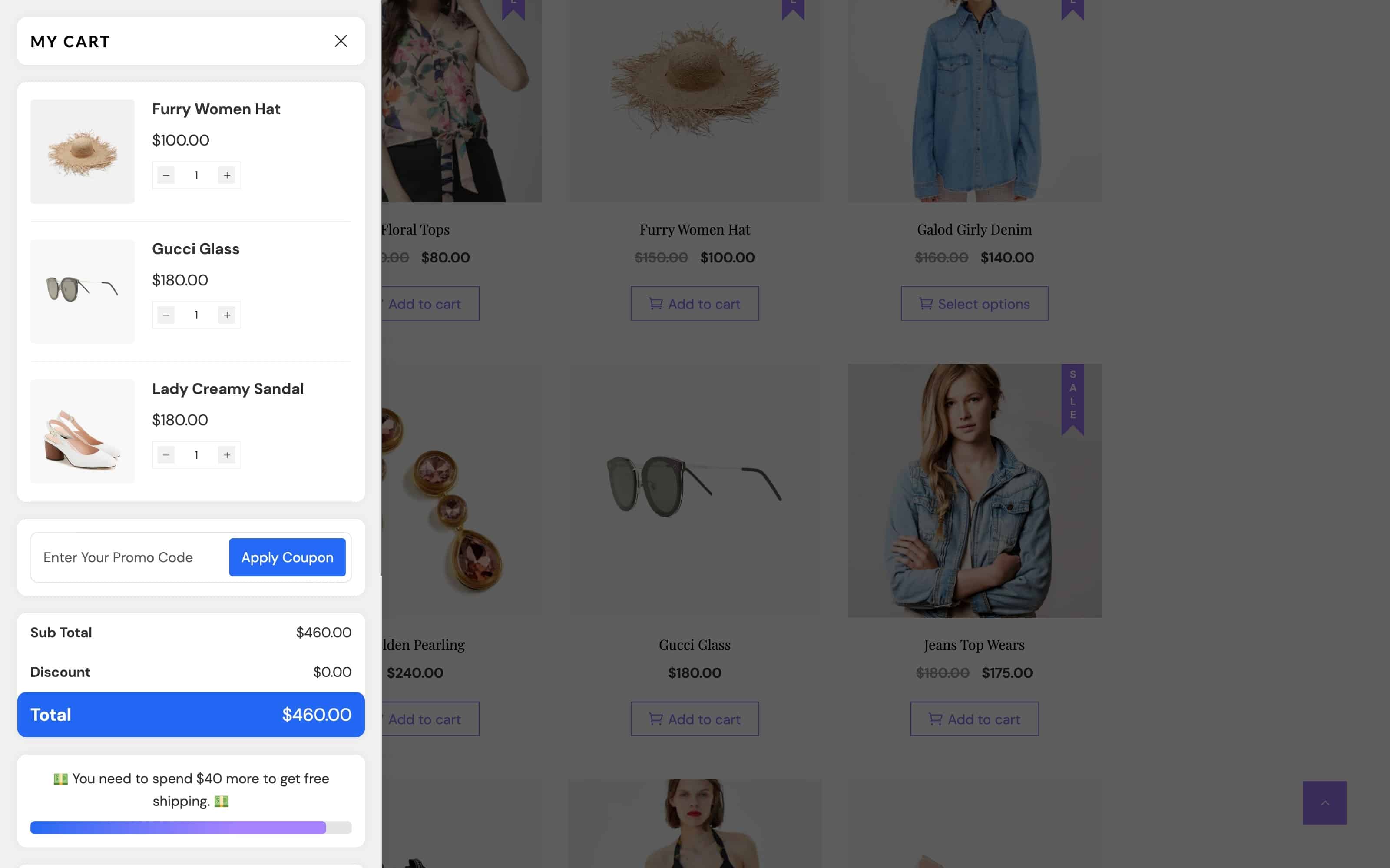The image depicts an online shopping cart and a feature showcasing several fashion items for women. On the upper left corner of the page, there is a "My Cart" section with an 'X' icon to close it. 

The cart includes:
1. A "Furry Woman Hat" accompanied by an image of a furry hat, priced at $100. A quantity selector allows for adjusting the number of items.
2. A pair of "Gucci Glasses" priced at $180, with a corresponding image and a similar quantity selector.
3. "Lady Creamy Sandals," also priced at $180, with a picture of white sandals and a quantity selector.

Following these items is a section labeled "Enter Your Promo Code" accompanied by a blue "Apply Coupon" button. Below this are the cart's financial details: a Subtotal of $460, Discount of $0, and Total of $460, displayed within a blue section. Additionally, there is a notification indicating, "You Need To Spend $40 More To Get Free Shipping."

On the right side of the page, there is a display of featured items including:
- "Galore Dirty Denim" priced at $140
- "Furry Woman Hat" priced at $100
- "Jeans Top Wear" priced at $175
- "Gucci Glasses" priced at $180

Images of women modeling these items, including clothing, glasses, and various ornaments, are visible, adding context and appeal to the highlighted products.